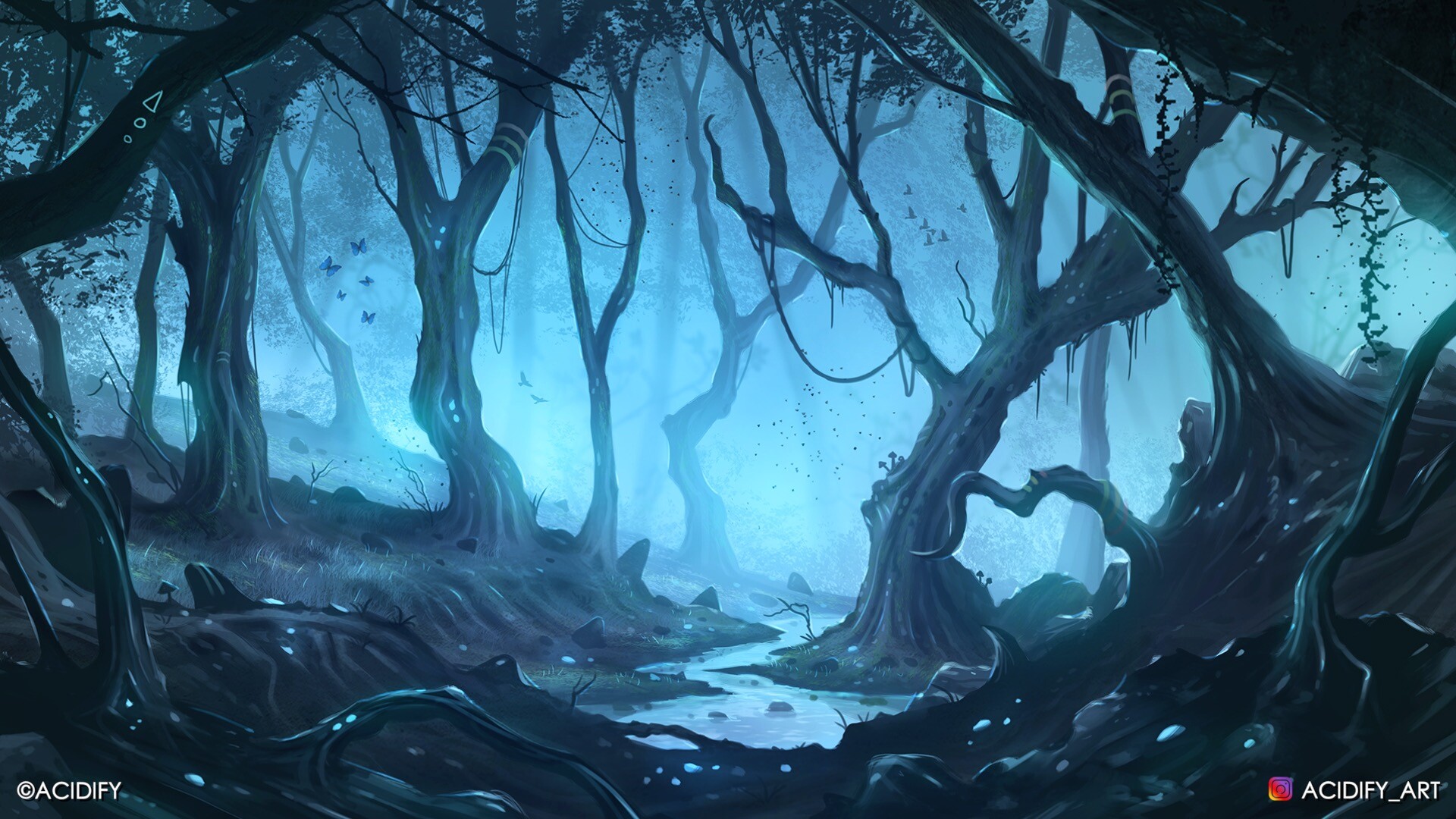This computer-generated, stylized image depicts a spooky, dark forest or swamp setting, characterized by a gloomy, moody atmosphere rendered in shades of blue, gray, and black. Dominating the foreground, a narrow stream zigzags through the center of the picture, flanked by dirt embankments. Twisted, gothic-style trees with dark gray bark reach unnaturally towards the sky, devoid of leaves and covered with vines and dangling ropes. These warped trees create an ethereal, surreal ambiance as their branches stretch and loop back in various directions. In the top left corner, there is a peculiar detail of a tree adorned with a white triangle and two white circles, reminiscent of butterflies or birds in flight. The image is tagged with "copyright ACIDIFY" in the lower left-hand corner and an Instagram link "ACIDIFY_art" in the lower right-hand corner, emphasizing its digital art origins. The entire scene invokes a sense of eerie unnaturalness, blending elements of forest and swamp in a hauntingly beautiful, stylized manner.